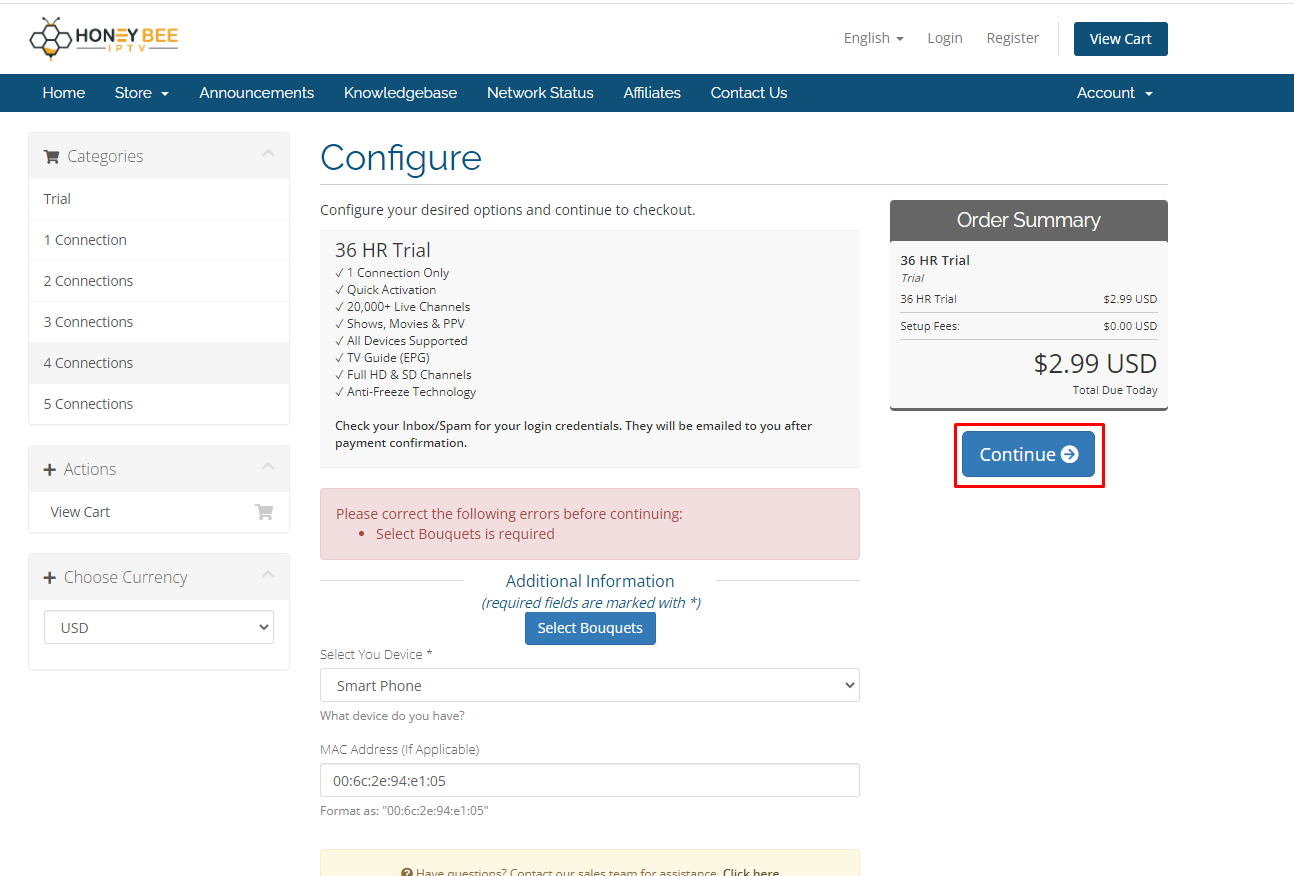The image is a screenshot from the Honeybee IPTV website, prominently displaying its interface and options for IPTV services. At the top-left corner, the Honeybee IPTV logo is visible, featuring a honeycomb design with the word "Honey" in black and "bee" in a bee-colored yellow, accompanied by "IPTV" in yellow.

The navigation bar at the top provides various options such as Home, Store, Announcements, Knowledge Base, Network Status, Affiliates, Contact Us, and Account. On the left side, there's a drop-down menu listing multiple subscription options: Trial, 1 Connection, 2 Connections, 3 Connections, 4 Connections, and 5 Connections. The "4 Connections" option is highlighted in gray, indicating it is currently selected. Below this, there's a section for Actions featuring a plus icon and a cart, with an additional option to view the cart. Further down, there's a drop-down menu for choosing the currency, set to U.S. dollars.

The central part of the screen shows a configuration section with the instructions "Configure your desired options and continue to checkout." The user has selected a 36-hour trial with 1 Connection, Quick Activation, access to 20,000 live channels including Shows, Movies, PPV, support for all devices, TV Guide, Full HD and SD, and Anti-Freeze technology. A note advises checking the inbox or spam folder for login credentials. There is a highlighted error message in pink stating, "Please correct the following errors before continuing: Select bouquets is required." Additional information requests the user to select their device, with a smartphone currently selected and the device's MAC address provided.

At the bottom, the order summary indicates a 36-hour trial for a fee of $2.99 USD, with the total amount due today. A red-highlighted "Continue" button is prominently displayed to finalize the order.